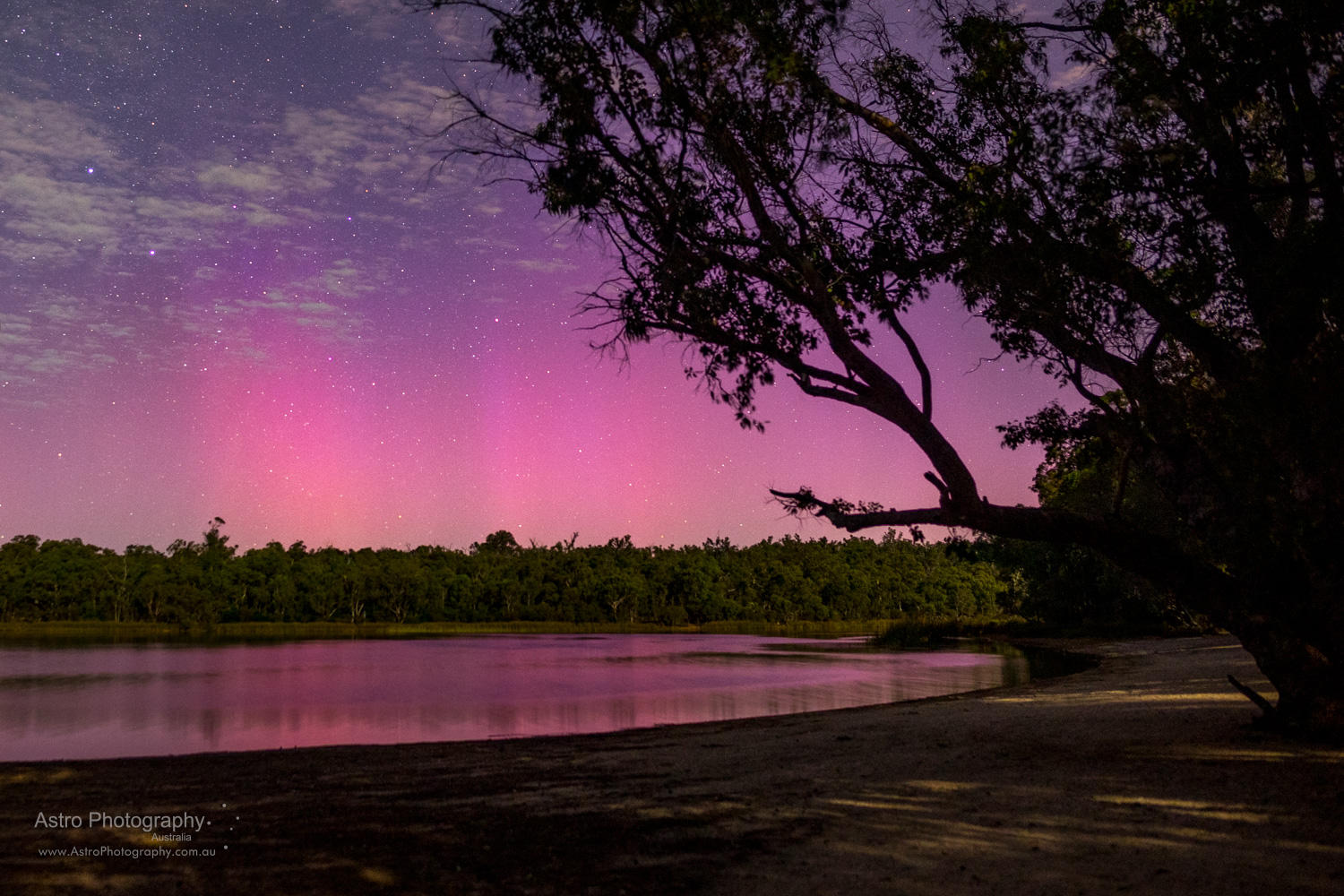This photograph captures a stunning evening scene featuring a purple and pink sky transitioning to light blue with streaks of gray clouds. Stars are visible twinkling above a serene body of water, likely a lake or large pond, bordered by a diverse landscape. In the far background, a dense row of green-leafed trees stretches horizontally, providing a natural frame. Dominating the right side of the image, a large silhouetted tree extends from the lower right corner upwards, its dark form stark against the colorful sky due to the lighting conditions. The foreground showcases a mix of dirt and grass with patches near the water's edge. The bottom left corner bears the watermark "astrophotography.com.au" in white text. Overall, the scene is a peaceful blend of natural elements set against the beauty of a transitioning evening sky and reflected light.